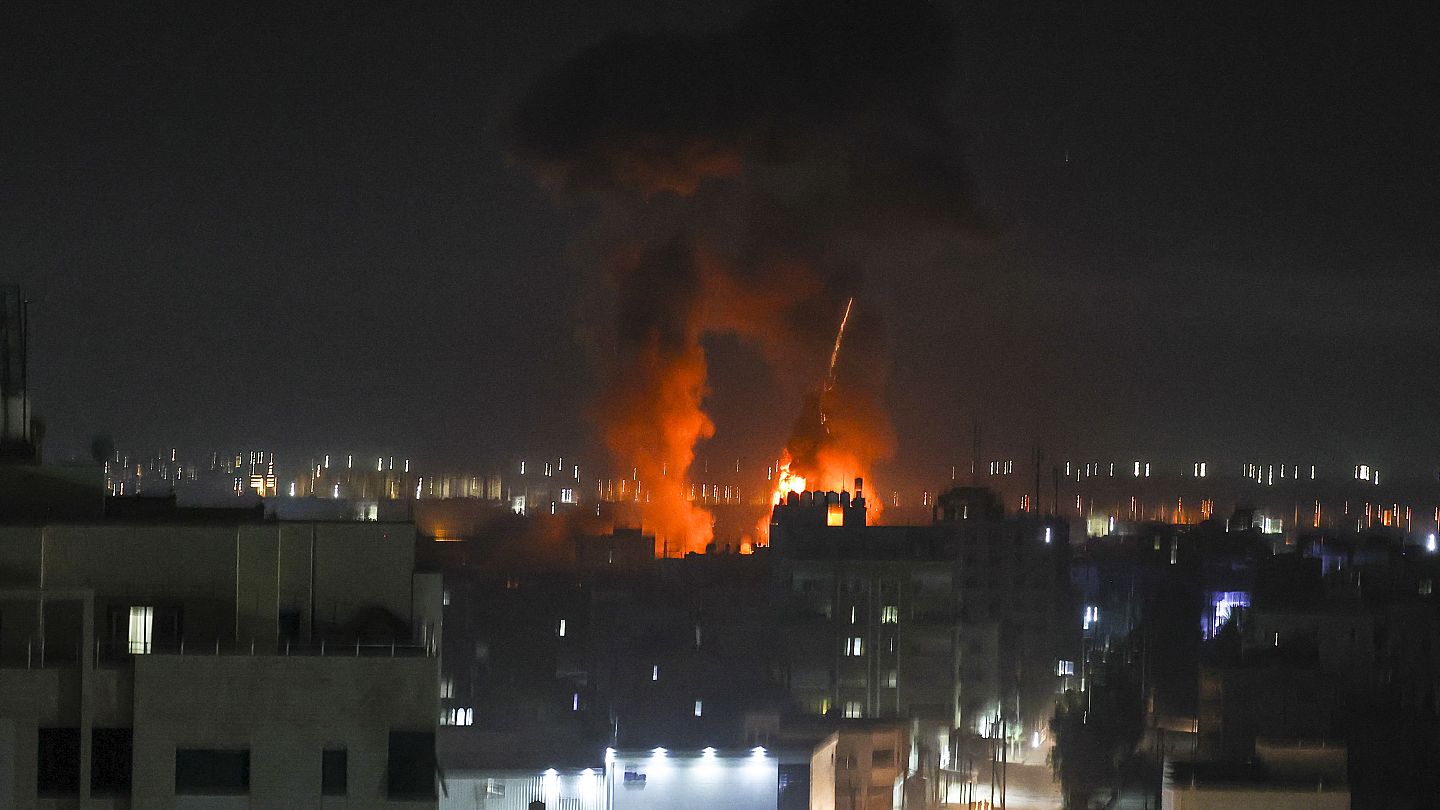This nighttime image of a city showcases a relatively low-rise urban landscape, with buildings maxing out at about 10 to 12 stories. Interspersed among these structures are various lights, both from within the buildings and from external sources, illuminating the scene. The photograph, though blurry and likely taken in a moment of urgency or panic, captures a vivid and alarming central feature: a bright orange fireball accompanied by plumes of thick smoke. The fire, possibly the result of a missile either launching or landing, burns intensely, casting an orange hue on the surrounding smoke that gradually darkens as it ascends, arching towards the top of the image. The sky looms dark and foreboding in the background, punctuated by indistinguishable lights far off in the distance. Despite the graininess, the impact of the fiery explosion in the heart of the image is unmistakable and dramatic.